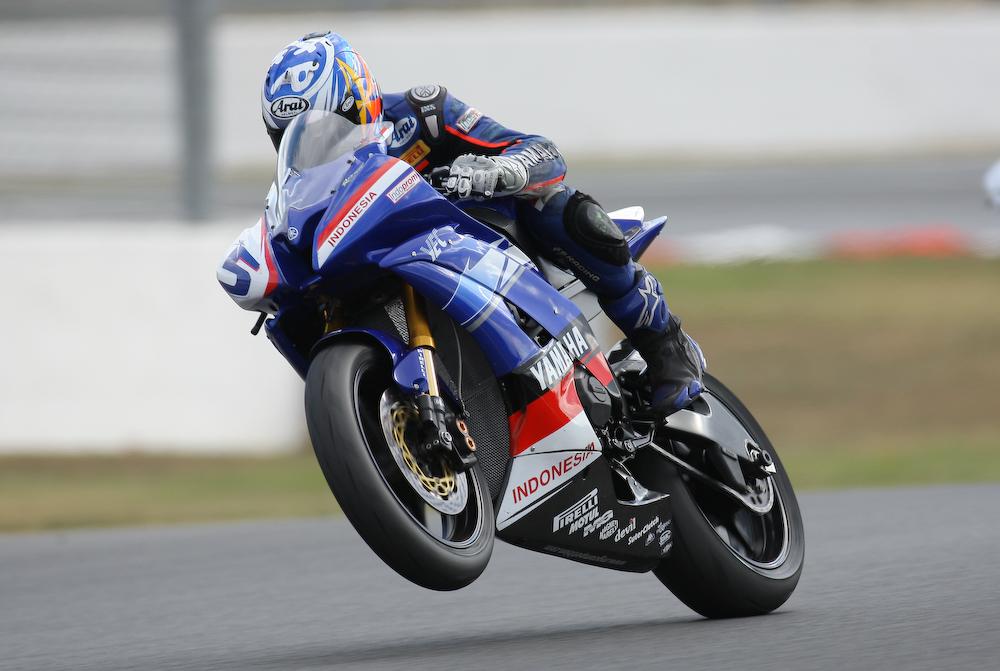This detailed caption is designed to be comprehensive and incorporates elements from each of the original captions:

---

This image captures a dynamic close-up of a motorcyclist in the midst of a race, performing a wheelie with the front wheel elevated at least six inches off the ground. The rider is leaning forward, dressed in a predominantly blue racing suit emblazoned with the Yamaha logo on the sleeve and a black buckle on the shoulder. Their white gloves and blue helmet, which bears the Arai logo at the front and colorful yellow and red flower-like symbols near the ears, complement the outfit. The motorcycle they are riding is primarily blue with red and white accents, marked notably with the word "Indonesia" on both the front and lower parts, along with the number 5. Adorned with logos from various sponsors including Yamaha, Pirelli, Trellis, Motul, and Devil, the bike emphasizes the racing context. The blurred background, featuring hints of green and a racetrack bordered in red and white, accentuates the high-speed action on the gray asphalt, highlighting the intense focus on the motorcyclist and their Yamaha bike.